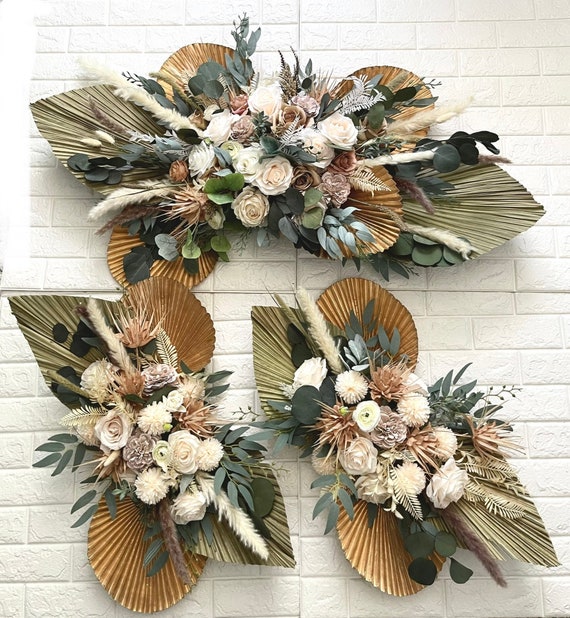The photograph depicts three meticulously arranged floral compositions mounted on a white brick wall. The top arrangement is larger, while the two at the bottom are smaller, yet all share a cohesive design. Each arrangement features a base of green leaves of varying shapes, from round to elongated, some large and colorful in tones of green and brown. Rising from the leafy base are clusters of artificial flowers in pale hues of white, light yellow, and light pink, accompanied by darker brown blooms. Among the flora, there are also tan or gold-colored clam shells, feathery white plants, white roses, and green plants adorned with berries, contributing to a harmonious color palette of green, gold, white, and pink. The consistent pattern of these elements across all three sets creates a visually appealing wall art display.